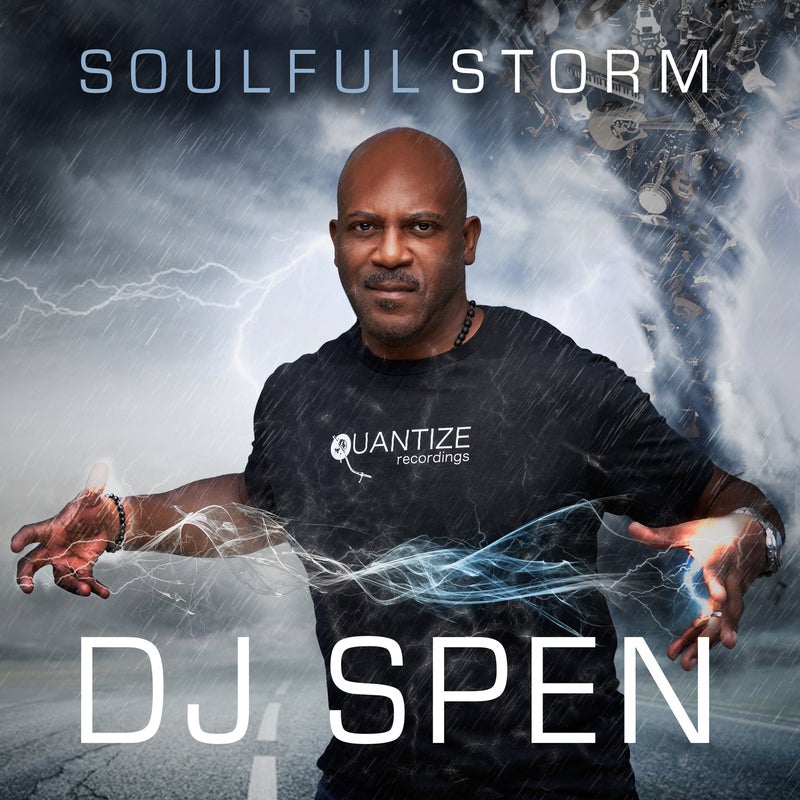The image depicts an African American man with a bald head and a mustache standing in the middle of a street amidst a dramatic stormy backdrop. He is wearing a black short-sleeved t-shirt with the words "Quantized Recordings" on his chest. The man, positioned centrally, extends his arms with his hands spread apart, and white lightning appears to emanate between them. The phrase "DJ SPEN" is prominently displayed below the lightning, all in capitalized letters. The scene is enhanced by a rainy atmosphere, with many musical instruments like guitars, drums, and a keyboard scattered in the background. A tornado swirls in the upper right corner of the image, contributing to the chaos of the black, lightning-filled sky. The title "Soulful Storm" is placed at the top of the poster-like image, which features a palette of black, gray, light blue, white, tan, and brown, giving it a moody and electrifying ambiance.